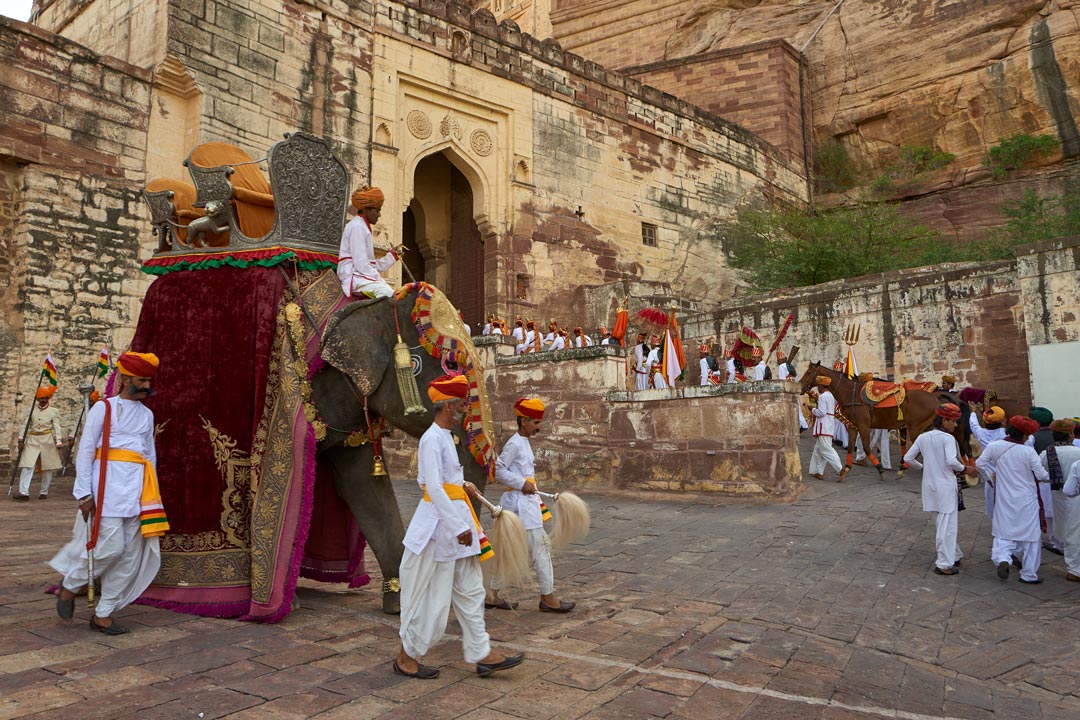The image depicts a lively outdoor scene featuring an elephant adorned with intricately decorated burgundy velvet cloths and gold tassels. A person clad in white attire topped with a turban is riding the elephant, which is surrounded by others in similar traditional white garments and turbans. Among them, some individuals also wear yellow belts and hats, adding a vibrant contrast. The gathering appears to be part of a ceremonial event, possibly of Middle Eastern or Indian origin, indicated by the attire and atmosphere. Numerous onlookers are present, contributing to the festive ambiance. In the backdrop, a brick building stands, while the upper right portion of the image displays elements of green, likely indicative of foliage or decor, enriching the scene's cultural and visual complexity.